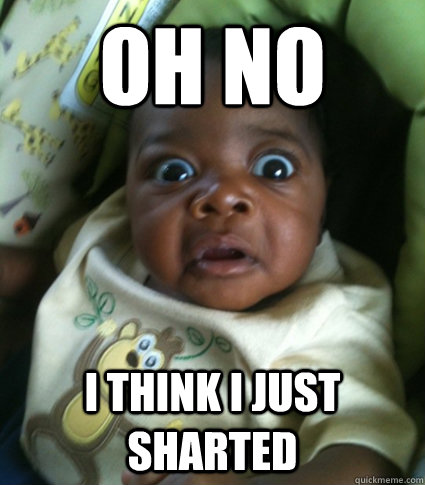The image is a striking, color photograph featuring a bald, muscular man with a lightly graying beard and visible chest hair. He's on all fours, leaning on a bed covered with a multi-colored comforter in shades of red, black, grey, and white. The man is nearly naked, wearing only some sort of black strappy underwear or shorts. Prominently displayed on his right shoulder is a round, black tattoo that vaguely resembles a bird's head. The bedroom around him is dark and moody, with black or dark grey walls and black leather pillows, some with white vertical stripes, positioned against a dark headboard. In front of him lies a black and white, cylindrical pillow partially obscuring his front. White text with a black outline spelling "H-A-I" appears at the bottom center of the image, resembling a greeting or meme. Additionally, there is small text at the lower right saying "quickmemes.com." The man gazes directly at the camera, creating a direct and somewhat provocative atmosphere.